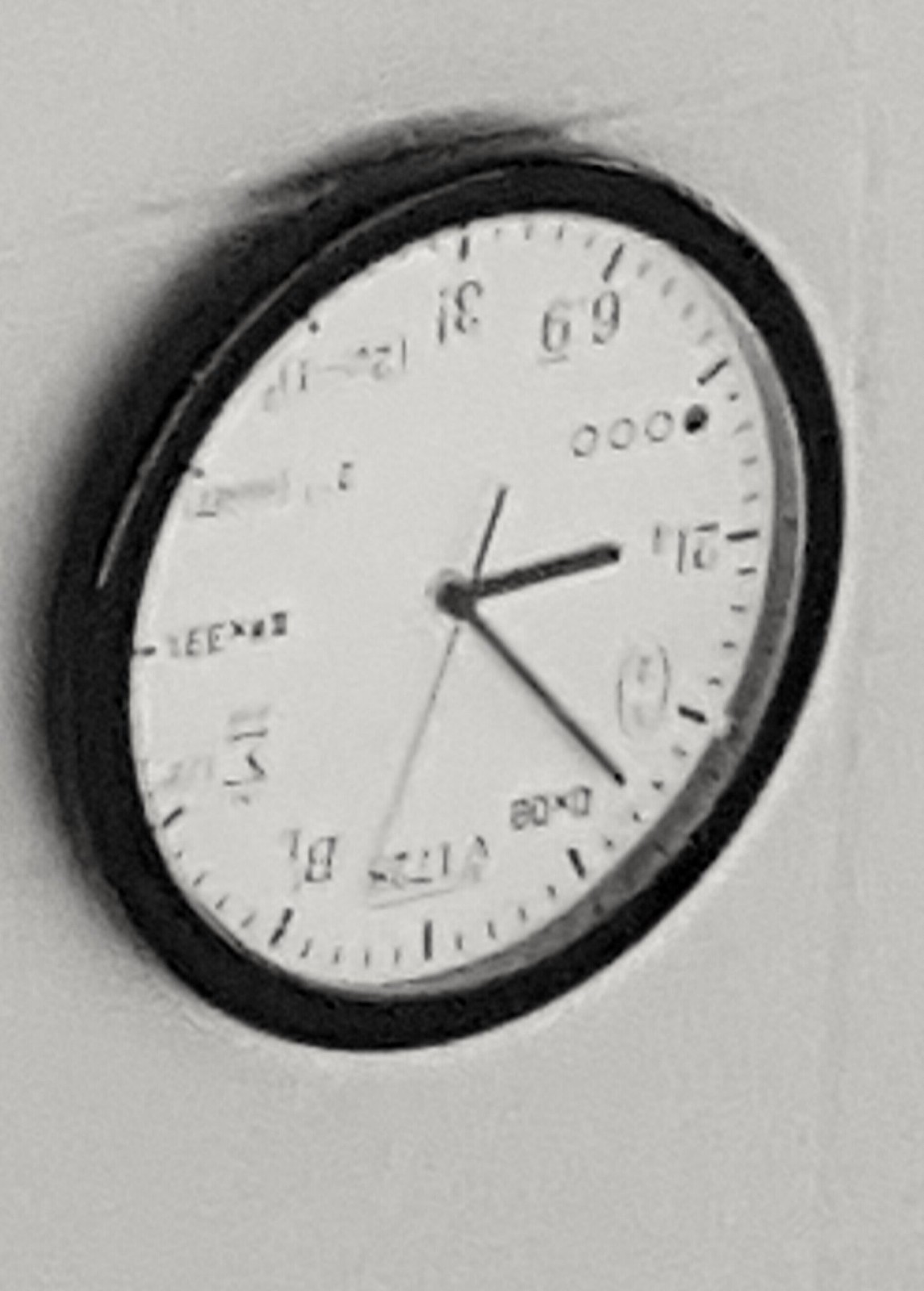This image is a vertical rectangular photograph of a blurry, grainy clock against a white brick wall. The clock, which has a black round frame and a white face, appears to be upside down. It is possibly encased behind acrylic or glass. The clock features black hour, minute, and long, skinny second hands. Instead of traditional numbers, the clock has various symbols and numeric representations. For instance, the position normally occupied by the number 7 shows a symbol resembling the Greek letter sigma, while the 8 position has the number 31 upside down and backwards (where the 6 would typically be). Other digits include mathematical symbols and unusual configurations like "3!" and "69" at different positions. This detailed yet disorienting arrangement of the clock's face gives it a uniquely offbeat appearance.